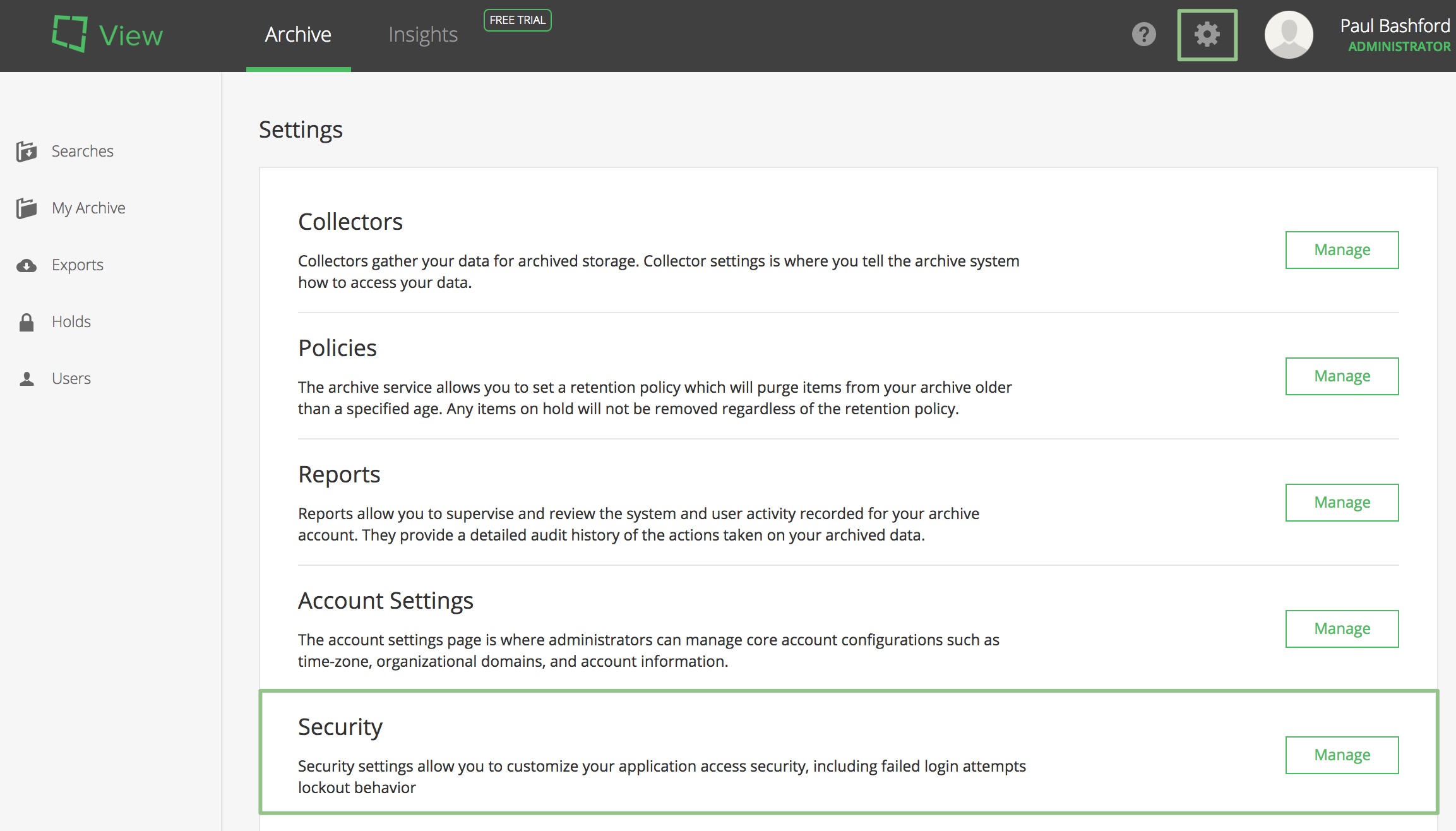This image captures a screenshot of a website interface. The top section features a dark gray horizontal bar, within which a green rotated rectangle showcases the word "View." Below this bar, the user has navigated to a section labeled "Archive," adjacent to a segment titled "Insights." A "Free Trial" button is prominently displayed at the top.

Additionally, the top navigation bar contains several clickable icons. The name "Paul Bushford" is visible, likely indicating the logged-in user. Below this, there is a panel with nested options including "Settings," "Collectors," "Policies," "Reports," "Account Settings," and "Security." Each of these options is housed within its own clickable gray rectangle.

The "Security" section is highlighted with a green border, indicating it is the currently selected option. To the right of this panel, there are several green rectangles labeled "Manage," which appear next to individual security settings, allowing users to configure these options further.